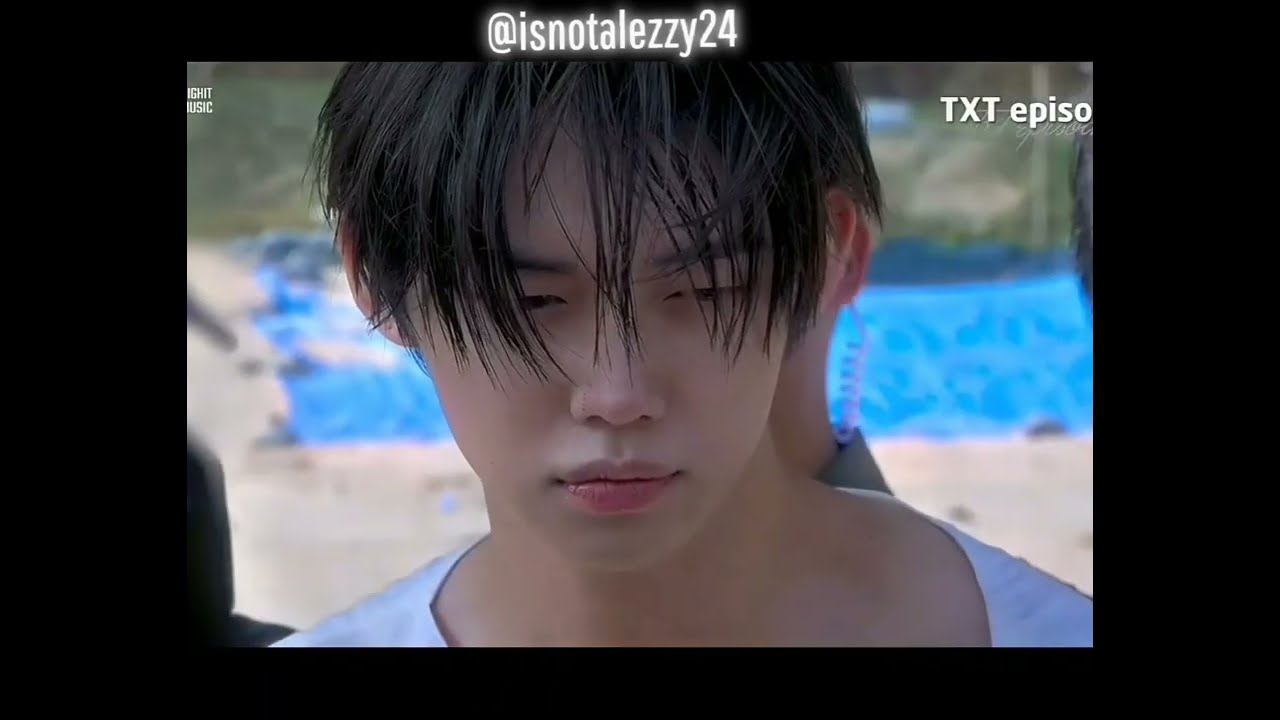The image depicts an Asian man with dark, slightly wet hair that falls over his eyes and reaches the tip of his nose. He appears to be looking down, not facing the camera directly, and has an expression that suggests he might be upset or troubled. He's wearing a white shirt with a somewhat stretched-out collar; the picture cuts off just below his neck, so the rest of his outfit isn't visible. The setting appears to be an outdoor scene near a pool, with a blurry blue pool in the background, framed by tan concrete and some greenery further back. Behind the man, there's another person with a Bluetooth earpiece, holding what could be a microphone or a speaker. The individual behind him partially obscures the background. The top of the image contains text in various colors, including tan, red, white, blue, light brown, green, and red. The text includes "@ISNOTALZ24" on the left and "TXT episode" on the right, though "episode" is cut off. Additionally, there's a black border around the photo.